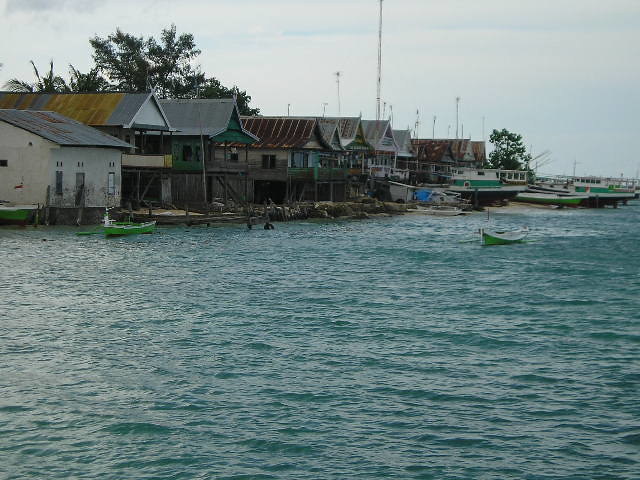This detailed image captures an overcast outdoor scene featuring a serene body of water, possibly a lake, river, or sea, with a hint of bluish-green hue and minimal wake. In the foreground, two small, unoccupied green boats float near the shoreline, anchored close to the water's edge. Nearby, a slightly larger green boat is tied to a dock in front of a cluster of old, Asian-style buildings characterized by their pointed, flared, rust-colored metal roofs. These buildings are tightly packed along the water's edge, each equipped with its own dock. Further into the background, larger boats rest on a sandy area. The sky is a mix of cloudiness with subtle patches of blue and hints of yellow. Scattered among the scene, one can observe tree leaves behind the houses and more trees in the distant background, adding a touch of nature to the overall setting.